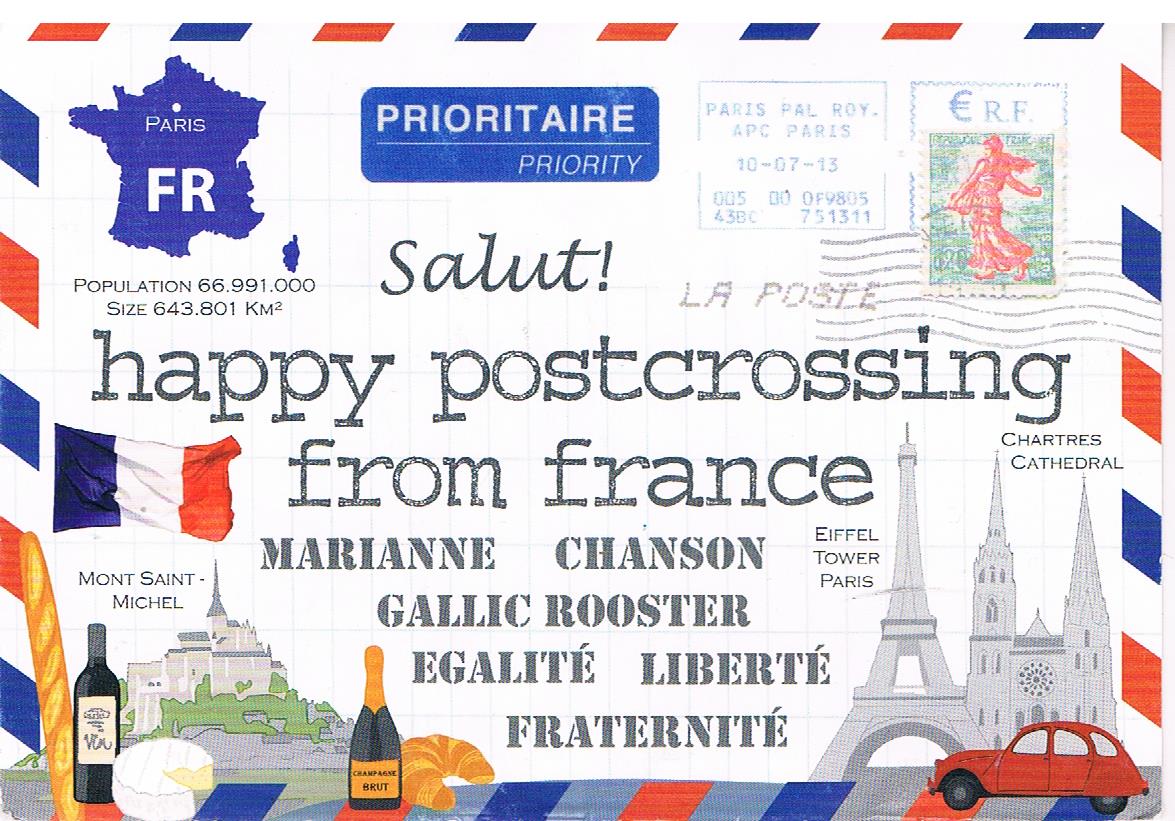This detailed postcard from France features a vibrant red, white, and blue striped border, echoing the French flag colors. The top of the postcard prominently displays the word "Salut" followed by "Happy post-crossing from France." It includes crucial information like "FR population 66,991,000" and "Size 643,801 km²." The upper left-hand corner features a blue map of France with a white dot marking Paris, accompanied by the label "Paris, France." Just above it, the terms "Prioritaire" and "Priority Mail" are noted, signaling its expedited mail status. Icons of French pride are scattered throughout the design, including the phrases "Marianne Chanson," "Gallic Rooster," and the French motto "Égalité, Liberté, Fraternité."

The bottom of the postcard is a visual celebration of French culture and landmarks. There’s an image of the Eiffel Tower, Mont-Saint-Michel, and Chartres Cathedral flanked by delicious French pastries like croissants and biscuits, along with bottles of wine and cheese. A small red car, likely French-made, adds a touch of everyday charm to the scene. Additionally, a French flag can be spotted in the lower left-hand corner, solidifying the postcard's nationalistic theme. The rich curation of iconic symbols makes this postcard a delightful showcase of France's cultural and historical landmarks.